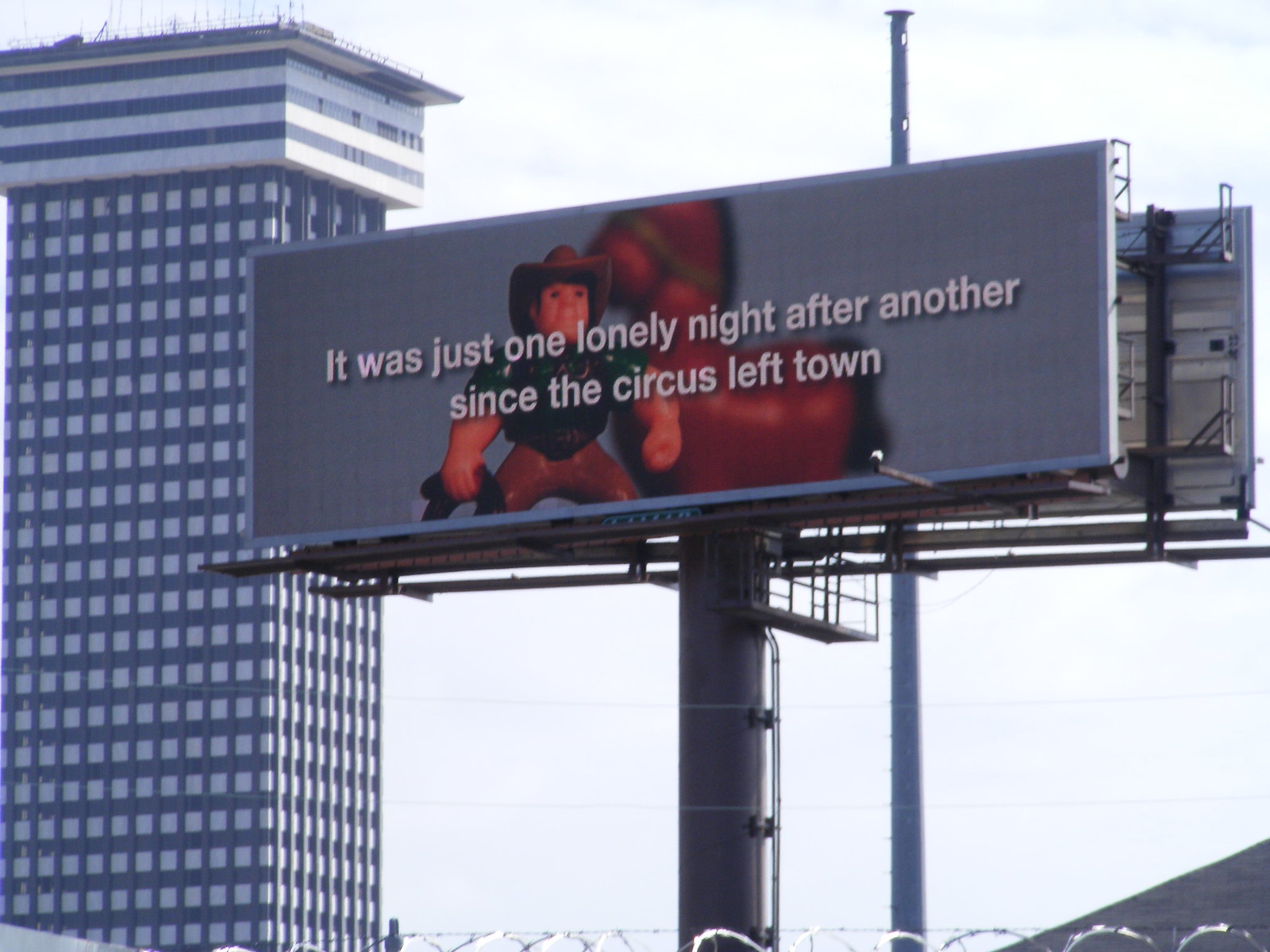The image depicts a cityscape dominated by a large billboard against an overcast sky, suggesting a dreary atmosphere. The billboard is supported by a greyish metal pole and displays the melancholic message, "It was just one lonely night after another since the circus left town," emphasizing a sense of abandonment and nostalgia. Prominently featured on the billboard is a plastic toy cowboy, squatting with a balled-up face and clutching something in one hand, donning a classic cowboy hat. A blurry plastic horse also appears in the background of the billboard image, adding to the scene's somber mood. Below the billboard, a wire fence with barbed wire runs horizontally, and a black post stretches vertically, intersecting the view. The surrounding environment includes a tall, grey, and white striped building, characterized by its rectangular windows, standing out against the cloudy, grey sky, which blends seamlessly into the subdued ambiance of the scene.